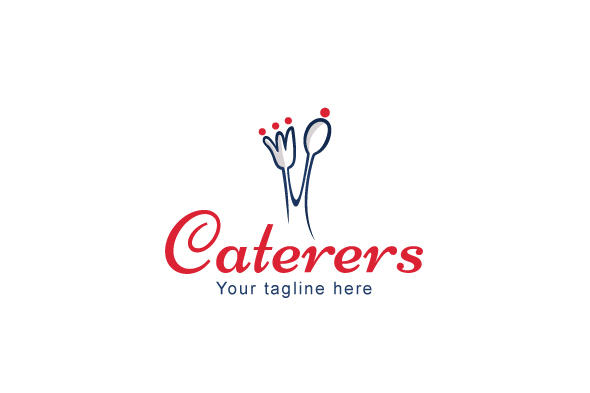The image depicts a stylized logo designed for a catering service. It features a fork and spoon illustration crafted in black line art that merges elegantly at the base, creating a single unified design. The fork has three tines, each topped with a red dot, and the spoon has an additional red dot above its bowl, making a total of four red dots. This graphic sits atop the word “caterers”, which is written in a red, flowing script font with rounded letters. Directly below “caterers” is the phrase “your tagline here” in a straightforward gray block style font. The entire logo is placed on a clean, white background, making the elements stand out distinctly.